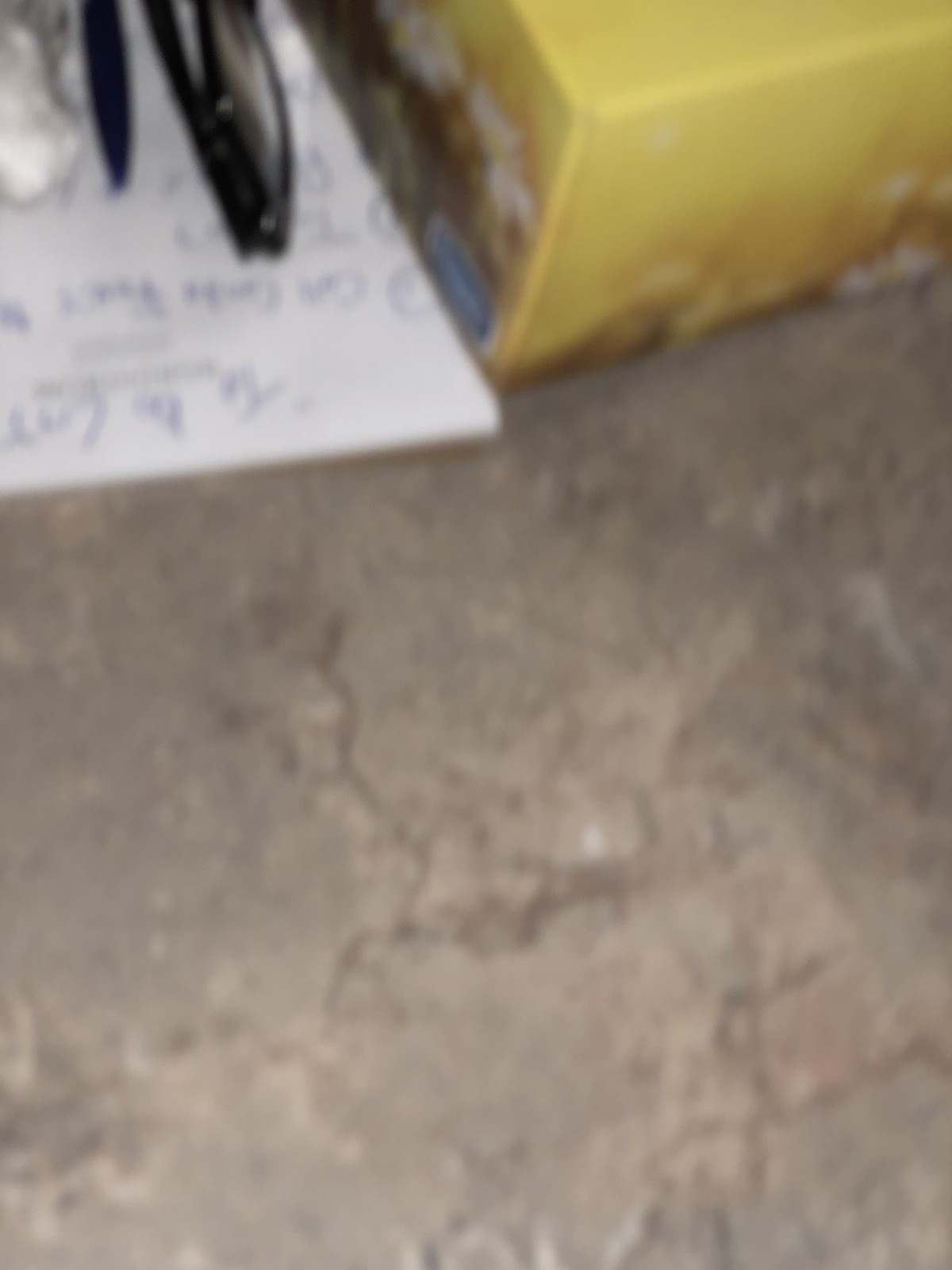The photograph showcases a granite or concrete countertop, occupying the majority of the image. In the upper quarter of the frame, a notepad rests with indiscernible writing due to the blurriness of the photo. Atop the notepad, a pair of glasses or sunglasses is clearly visible. Adjacent to the notepad, there is a small, rectangular, yellow box that shows signs of dirt or rust along its bottom edges. The box is wider than it is tall and features a blue logo on it. The remainder of the photograph highlights the expanse of the countertop surface.